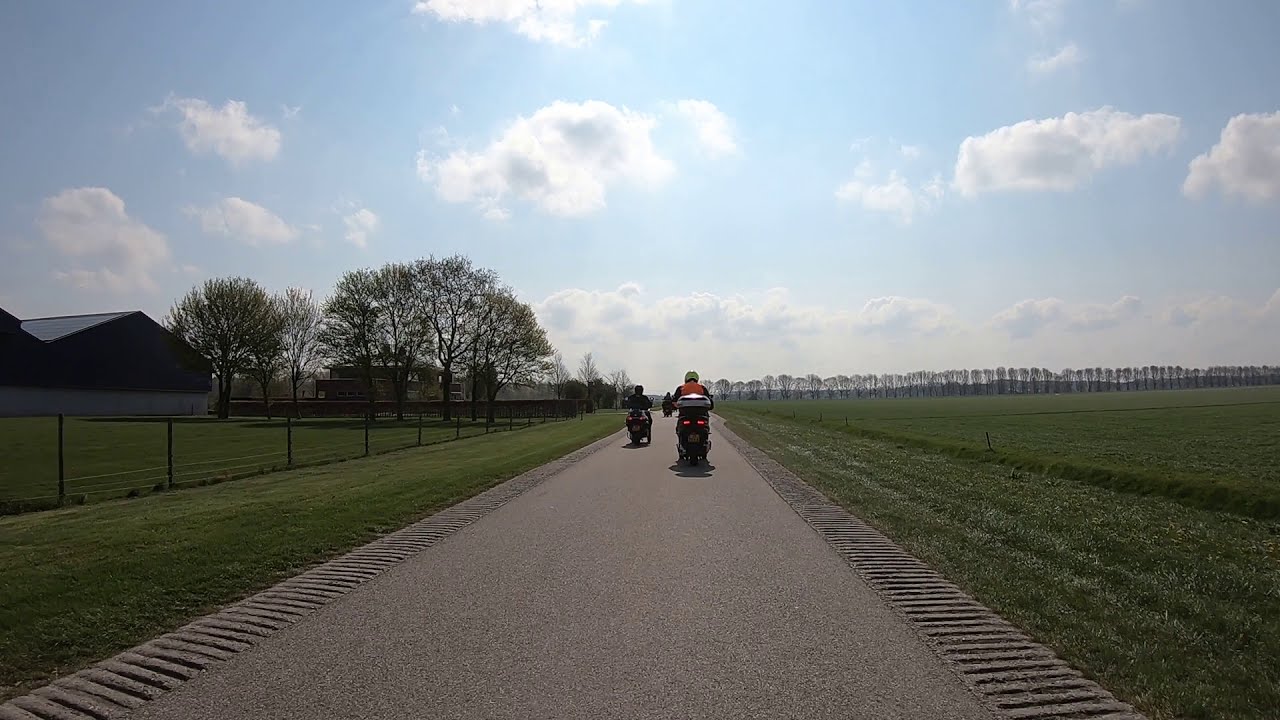The image showcases a narrow, single-lane countryside cement road extending straight from the foreground to the background. The road is flanked by ridges marking its edges. To the right, a vast green field stretches out, punctuated by a distant row of trees under a blue sky with scattered white clouds, indicating it's daytime. On the left, a small green grassy area leads to a short black chain link fence which encloses a larger field. Beyond this field, a grey and white building with a triangular roof can be seen, as well as another similar building further in the background. The road hosts several motorcyclists traveling away from the viewer, with three clearly visible. The foremost motorcyclist rides a black motorcycle with a white cargo area, wearing a distinctive yellow helmet and a blue and orange jacket.